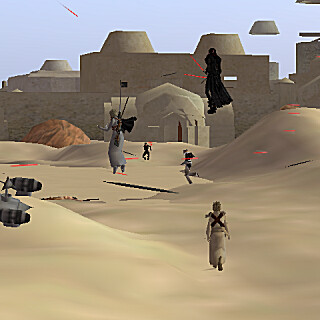This image, seemingly a screen grab from a video game with a Star Wars theme, portrays a dramatic desert scene. The terrain features tan, hilly dunes interspersed with patches of gray. Dominating the foreground is a character seen from the back with an X-shaped mark, while further back, a couple of figures are running toward a distant fortress structure under a light blue sky. A woman with a long braid and an angel wing, dressed in a gray gown, appears to be flying, and near her, a large black figure—presumably Darth Vader—levitates menacingly with two red lightsabers in hand, emitting red rays or bombs. Additionally, the left-hand side of the image shows what looks like the end of a gun or the engines of a war machine, suggesting an ongoing battle, as highlighted by red laser dashes streaking across the scene.